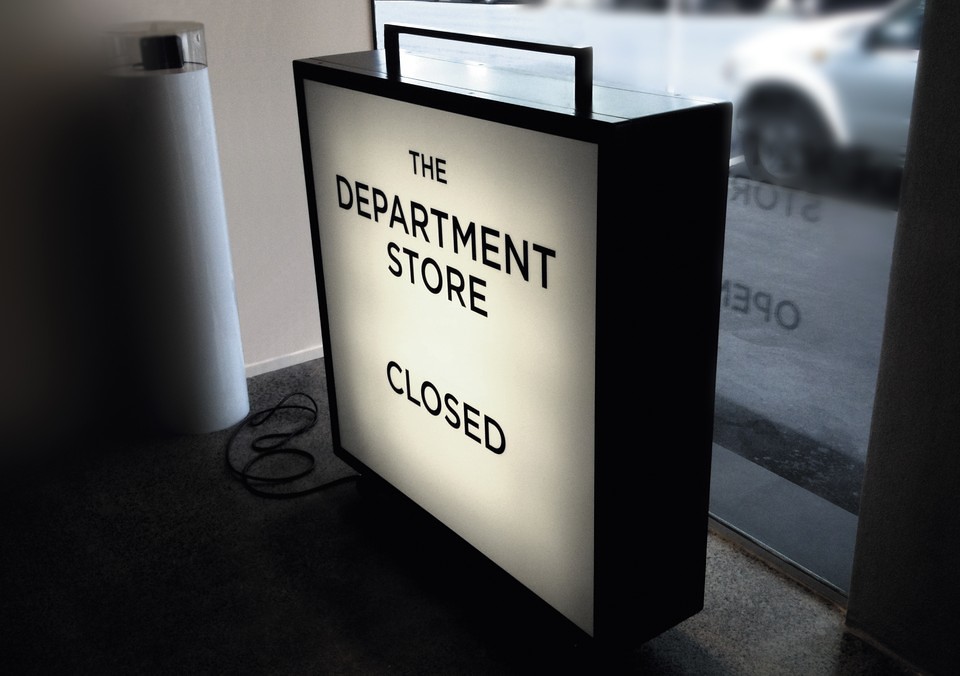The photograph captures an indoor scene featuring a prominent sign in a department store. The sign is a large, square, box-like structure positioned in front of a window that looks out onto a city street. It is backlit and displays the message "The department store closed" in black lettering on a white background. The window, slightly dirty, also reflects the word "open" from the other side of the sign, indicating that it can be flipped to show whether the store is open or closed. The sign has a handle at the top and a power cord plugged in at the bottom left, suggesting it is either an LCD sign or illuminated by the internal light.

To the right of the sign, there is a grey curtain and just beside it, a white car is visible parked on the street outside. Inside, the room features a dark gray carpet and beige walls. Adjacent to the sign on its left, there is a tall, cylindrical wastebasket with a silver top. Overall, the scene is well detailed with various elements contributing to the everyday ambiance of a department store interior.